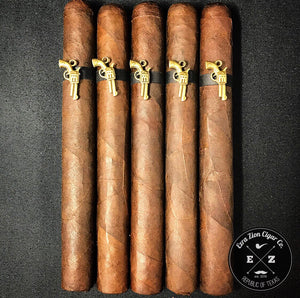The image shows five brown cigars laid out in a row on a dark, textured surface. Each cigar features a black band positioned near the top, adorned with a gold revolver icon, its barrel pointing downward. In the bottom right corner, a logo in a circular design reads "Ezra Zion Cigar Co." with the text "Republic of Texas" below it. Inside the circle, there is a cross design separating a pipe, an E, a Z, and a mustache in each quadrant. The overall dark background contrasts with the cigars and enhances the detailed gold and black elements in the image.